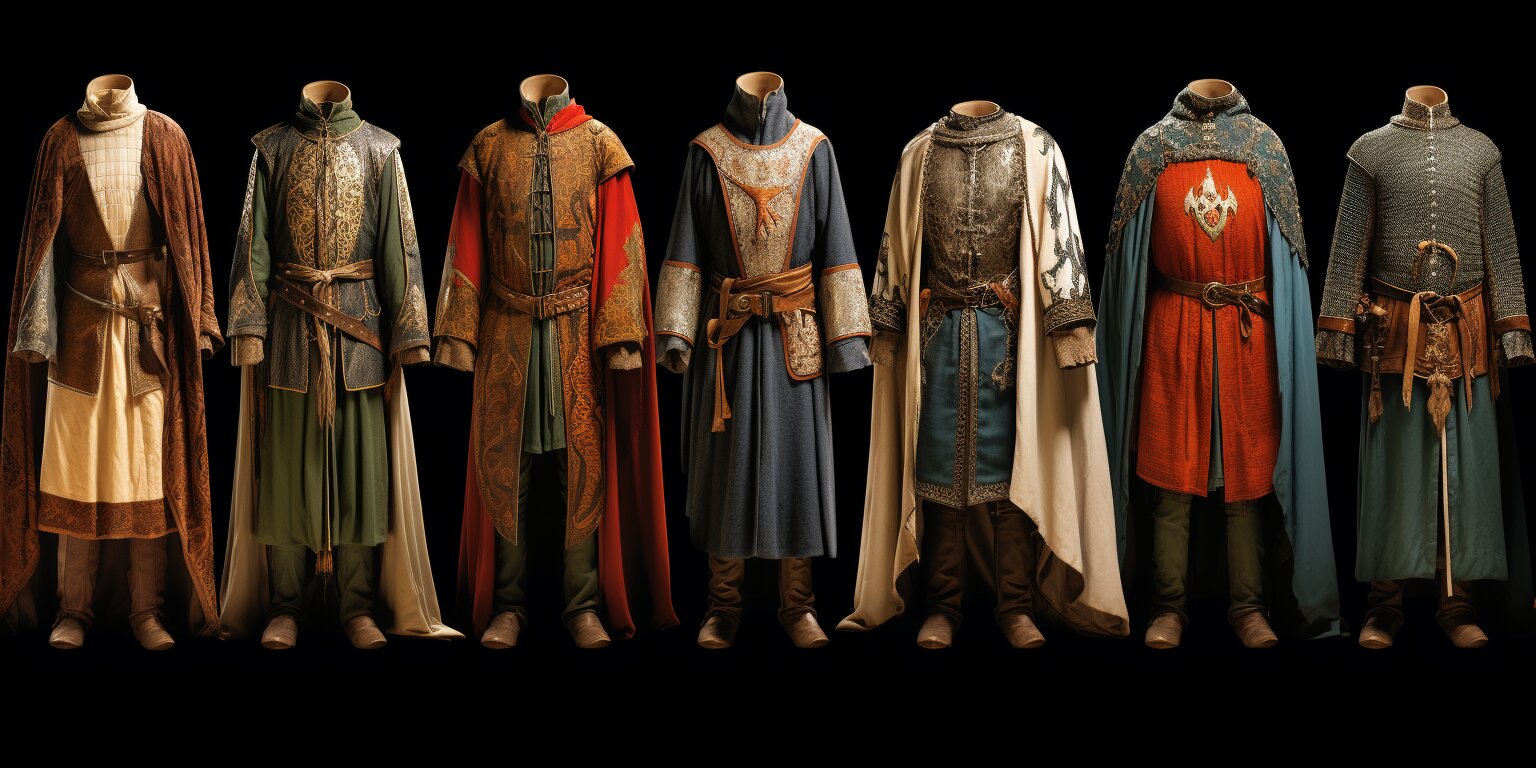Against a black background, the image displays seven examples of medieval men's clothing, each ensemble meticulously detailed down to the boots. These garments, which harken back several hundred years, appear animated but headless, standing as if worn by invisible figures. The outfits, showcasing a variety of colors and patterns, include tunics, robes, and layered ensembles, each accessorized with leather belts and brown boots. 

From left to right, the first outfit features a brown robe over a cream gown, paired with pants. Next is a green and blue attire followed by a brown and red ensemble. The fourth, centrally positioned outfit, displays blue and gray shades with silver accents. Moving right, the fifth outfit combines white, gray, and blue, while the sixth presents a mix of red, blue, and olive. Finally, the rightmost outfit features a distinctive upper part made of silver, a leather belt, and a skirt-like section above a blue lower part. An element of visual intrigue is added by the rightmost figure, who appears to have a sword fastened at the side. All figures lack heads and hands, focusing attention entirely on the elaborate medieval designs.